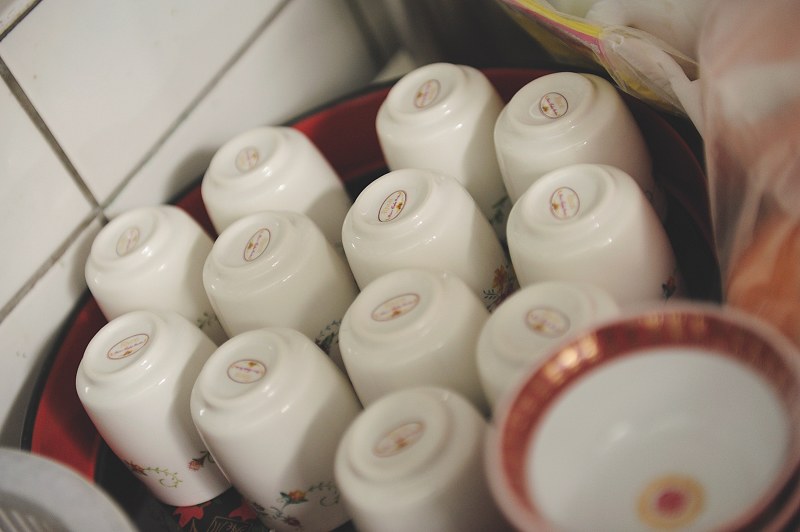The image features a diagonally downward view of a round, red plastic container filled with twelve upside-down, off-white tea or coffee cups. Each cup has a red oval with writing on the base, although the writing becomes blurry towards the lower right side. To the left of the cup-filled container is an off-white tiled wall with rectangular horizontal tiles and gray grout. In the lower right corner, there's a small glass bowl with a dark red rim and a decorative pattern reminiscent of those found in Chinese restaurants. Additionally, the setting appears to be a kitchen area, as suggested by the background elements such as white drawers or cabinets and plastic storage bags.